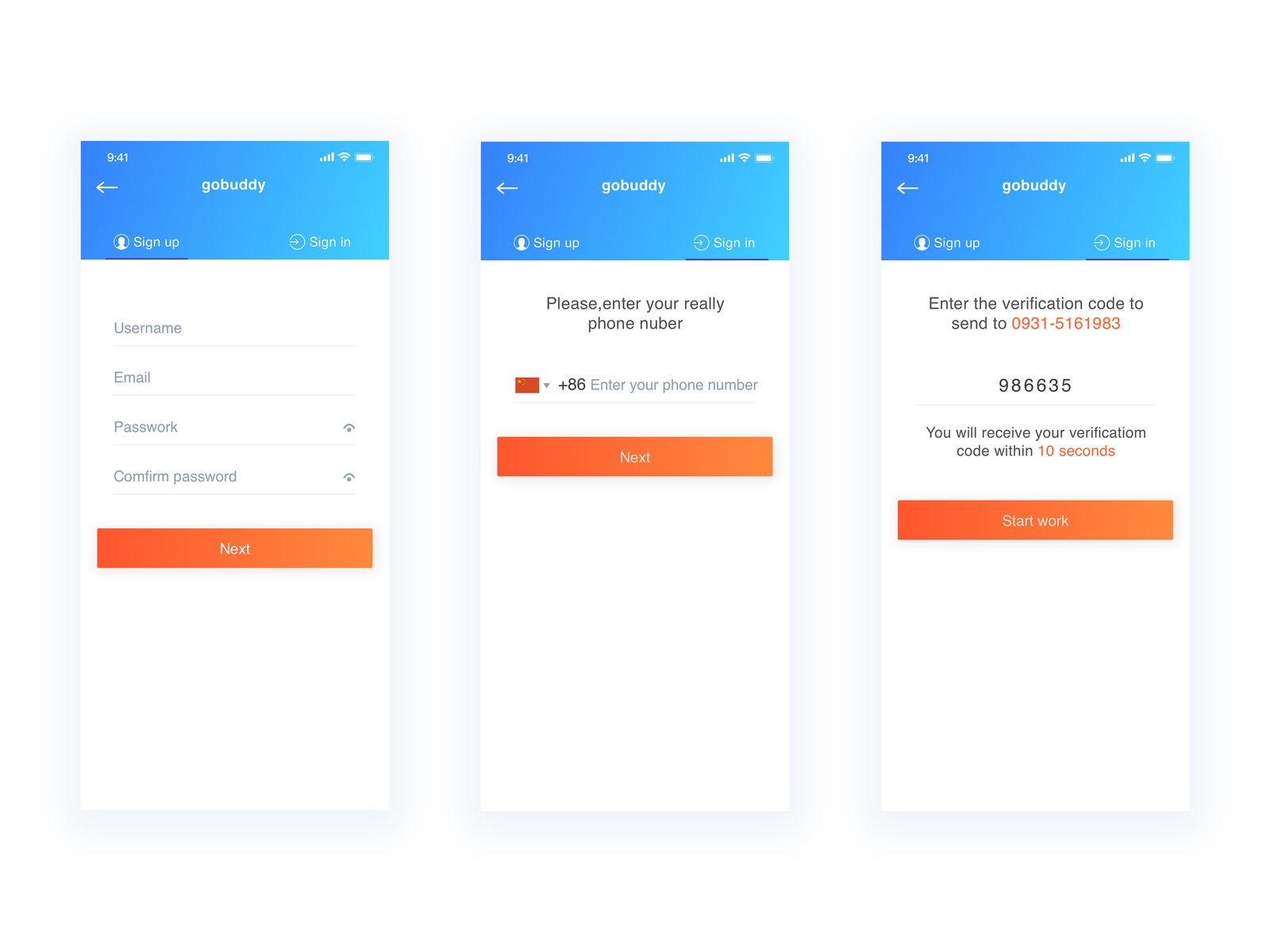The composite image features three screenshots captured from a smartphone, each showcasing different stages of the GoBuddy application's user authentication process. The status bar remains constant across all three images, displaying the time as 9:41 in the top-left corner, accompanied by battery, Wi-Fi, and signal strength icons on the top-right. The application operates on a blue background, except for specific interactive sections highlighted in white.

**First Screenshot:**
This image depicts the "Sign-Up" page of the GoBuddy app. At the top of the screen, "GoBuddy" is prominently displayed in white, set against the blue backdrop. A white, left-pointing arrow is positioned to the left of the app's name. Below the app's name, there are two tabs: "Sign-In" and "Sign-Up," with "Sign-Up" currently selected. The sign-up form includes fields for entering a username, email, password, and confirming the password. At the bottom, there is an orange "Next" button to proceed.

**Second Screenshot:**
The central screenshot transitions to the "Sign-In" page. Similar to the first, the name "GoBuddy" and the white arrow remain at the top. This time, the "Sign-In" tab is highlighted. The page prompts users to "Please enter your real phone number" twice due to a typographical error. It further displays an international dialing code (+86) and provides a field for entering the phone number. An orange "Next" button is present at the bottom, consistent with the sign-up page.

**Third Screenshot:**
The final screenshot continues within the "Sign-In" process. The user is prompted to enter a verification code, with the instruction "Enter verification code sent to 09315161983" placed prominently. The code received, "986635," is already populated in the field. A note below assures users that the code will arrive within 10 seconds, with "10 seconds" highlighted in yellow. The orange button at the bottom now reads "Start Work," replacing the usual "Next."

This detailed visual walkthrough of the GoBuddy app's user sign-up and sign-in stages aims to provide clarity and assist new users in navigating the authentication process effectively.